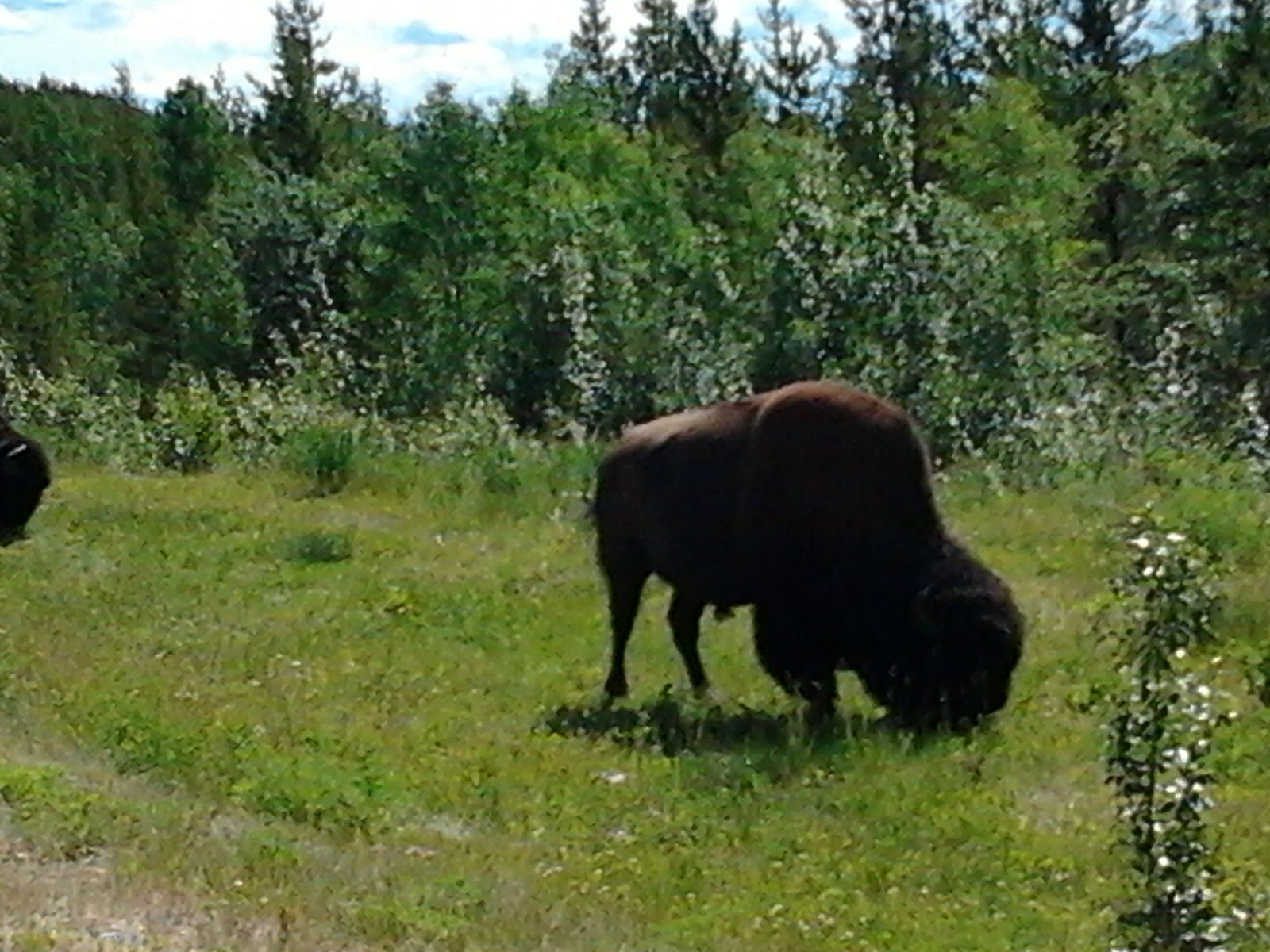In this photograph, a large buffalo is prominently positioned just right of center, bending its head down to graze on the lush green grass of a sprawling field. The buffalo's body is primarily a brownish color, with its head appearing darker, almost black. To the bottom left of the image, a bit of gravel hints at a nearby path, while a plant emerges in the foreground on the bottom right. Behind the buffalo, the field transitions into taller grass and weeds, which then give way to a dense line of leafy green trees stretching across the entire background beneath a sky dotted with some clouds, suggesting a bright and sunny day. Subtly, at the very left edge of the frame, the partial head of another buffalo is visible, peeking in from outside the main scene.